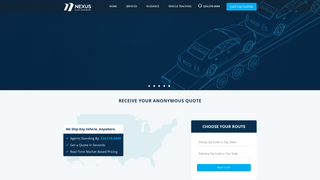The image features a blue banner at the top with white text that reads "Nexus," though the writing is slightly difficult to discern. Below the banner is a photograph set against a bluish background, capturing a long tow truck transporting two cars arranged bumper to bumper. The truck is visible with three of its wheels clearly showing, indicating its extended length. In this image, there is a noticeable space at the rear of the truck, emphasizing its capacity. Additionally, the image includes a small caption stating, "Receive your anonymous quote," along with further information that is quite small and challenging to read. Five dots are visible around the image, possibly indicating a sequence or additional navigation options. The word "Nexus" is further highlighted by two white lines flanking the letter "N," enhancing its visibility. Overall, the picture visually conveys the service of vehicle towing provided by Nexus.